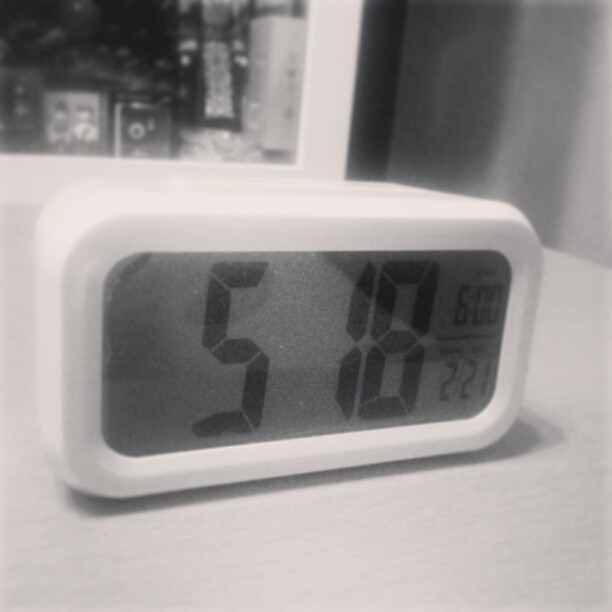This black-and-white photograph, slightly blurred and of low resolution, features a close-up of a digital clock encased in white plastic with rounded edges. The rectangular clock displays the large black numbers "518" prominently on its gray face. Above the time, a smaller "600" likely indicates a set alarm, while below, "2.21" appears to denote the date. The clock rests on an almost white, textured surface. In the background, a window or the edge of a cupboard framed in white is visible in the upper left-hand corner, containing what seem to be jars or metal objects. To the right, a greyish, textured area with varying shadows could be curtains. A shadow cast by the clock to the left adds depth, while the overall grayscale tonality suggests that the entire scene is devoid of color, enhancing the focus on the clock itself.